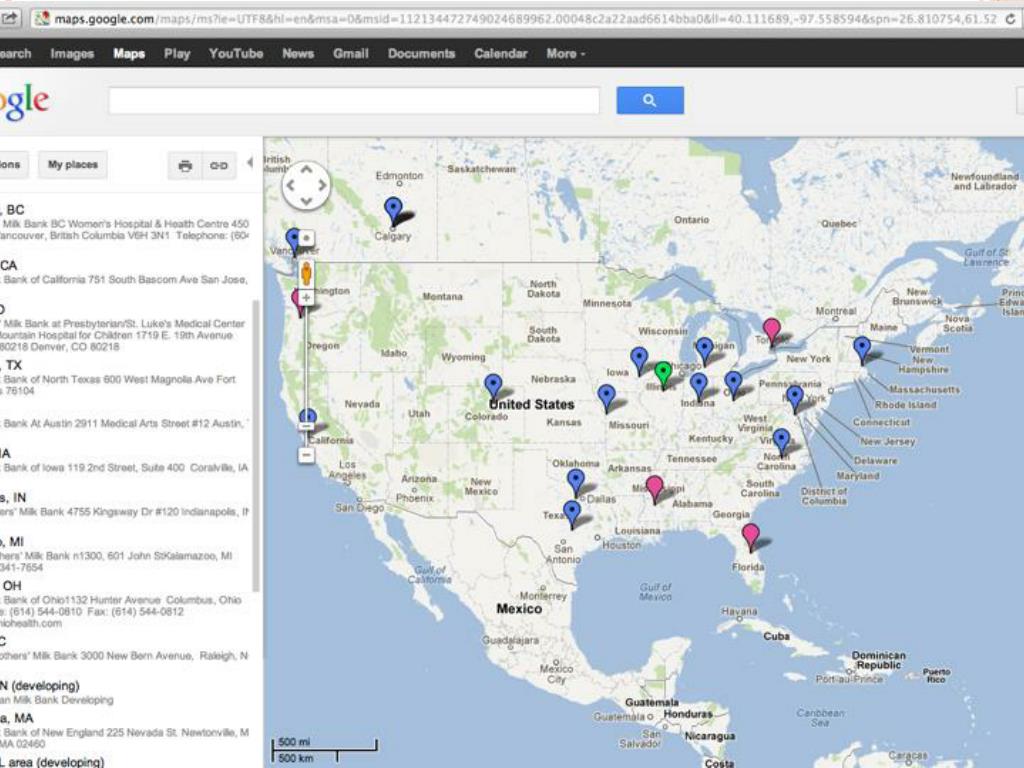The image displays the Google Maps homepage. In the upper left corner, there is an icon of a box with an arrow pointing to the right. Adjacent to this, a search bar is present, featuring the Google Maps logo and the address "maps.google.com" followed by the rest of the URL. On the far right of the address bar, a refresh icon is visible. 

Below the address bar, a black navigation banner extends across the screen. Although partially cut off on the left, the banner likely reads "Search," followed by "Images," "Maps," "Play," "YouTube," "News," "Gmail," "Documents," and "Calendar," ending with a "More" option accompanied by a dropdown arrow. 

Farther down, the top left corner of the Google logo is partially cut off. To its right, there is a search input area, and next to it, a blue rectangle containing a magnifying glass icon, indicating the search button. 

The main section of the screen displays a map highlighting the United States, along with parts of Canada and Mexico. Various location icons are scattered across the map in red, green, and blue, with blue being the predominant color. A single green icon is notably around Illinois. To the left of the map, some text provides information about states, but this content is also truncated and not fully visible.